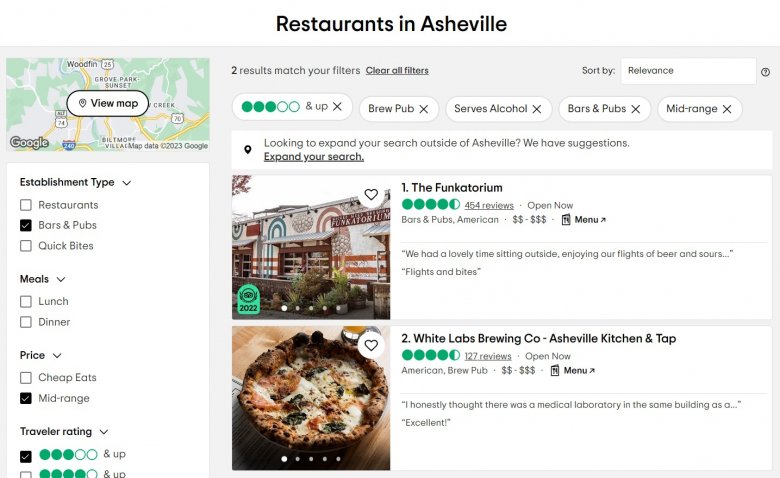The image displays an application that enables users to search for various types of places such as restaurants, bars, and quick-bite spots. The interface features a small map located in the top left corner. Below the map, there are several search criteria options available for user specification. In this particular search, the user has selected criteria for bars and pubs with a mid-range price level and ratings of at least three stars.

The search results present two specific establishments. The first result is "The Functorium," which boasts an impressive 4.5-star rating. The accompanying picture shows the exterior of the establishment. The second result is "White Labs Brewing Co, Asheville Kitchen and Tab," which also has a 4.5-star rating but with fewer reviews—127 compared to The Functorium's 454 reviews. The image for this result displays a sample meal from the establishment.

Overall, the application provides a clear, visual representation of matching venues based on the selected criteria, helping users make informed choices about where to go.